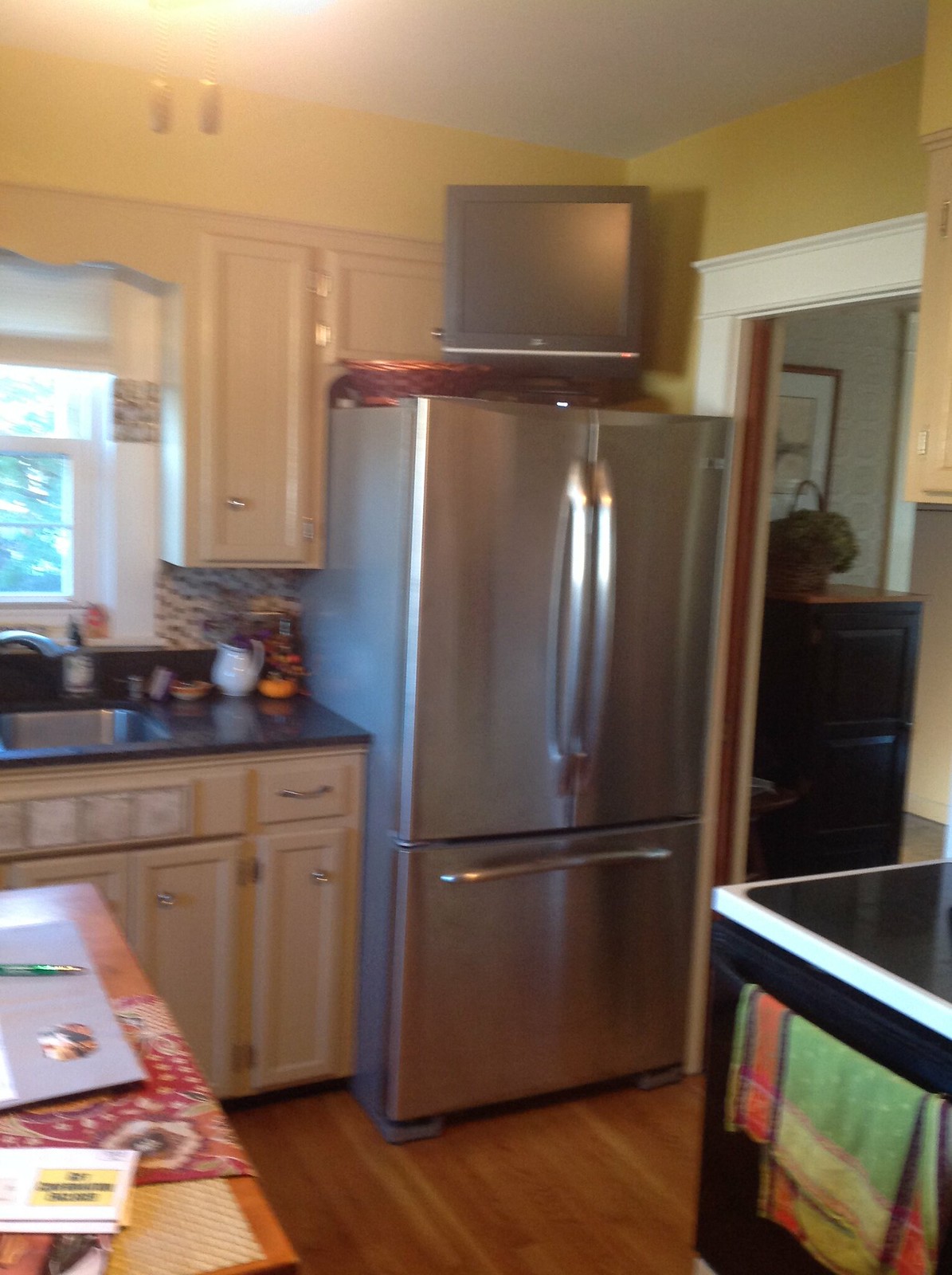The photograph depicts a modern farmhouse-style kitchen with various details centered around a prominent double-door, bottom-load stainless steel refrigerator. Atop this refrigerator is a small, approximately 48-inch TV. To the right of this unit is a doorway, marked by white molding, leading into what appears to be a dining room. The top of the walls are painted lemon yellow, contrasting with the white ceiling.

To the refrigerator's left, white cabinets are adorned with a black marble countertop, which houses a sink beneath a wall-mounted cabinet and a small window, allowing some natural light to filter in. The floor is made of light maple wood, which extends throughout the room.

The bottom right corner of the image shows a black stovetop with white edging, over which a green and yellow towel is folded. In the center, there's a cooking island that matches the maple flooring. Various small dishes and vases are neatly stacked along the backsplash of the countertop.

Adding to the kitchen’s detailed layout, a blurred wooden table with mail and a pen on it sits in another unspecified area within the image. The overall setting is illuminated by a bright ceiling light, with a slightly out-of-focus quality to the photograph.